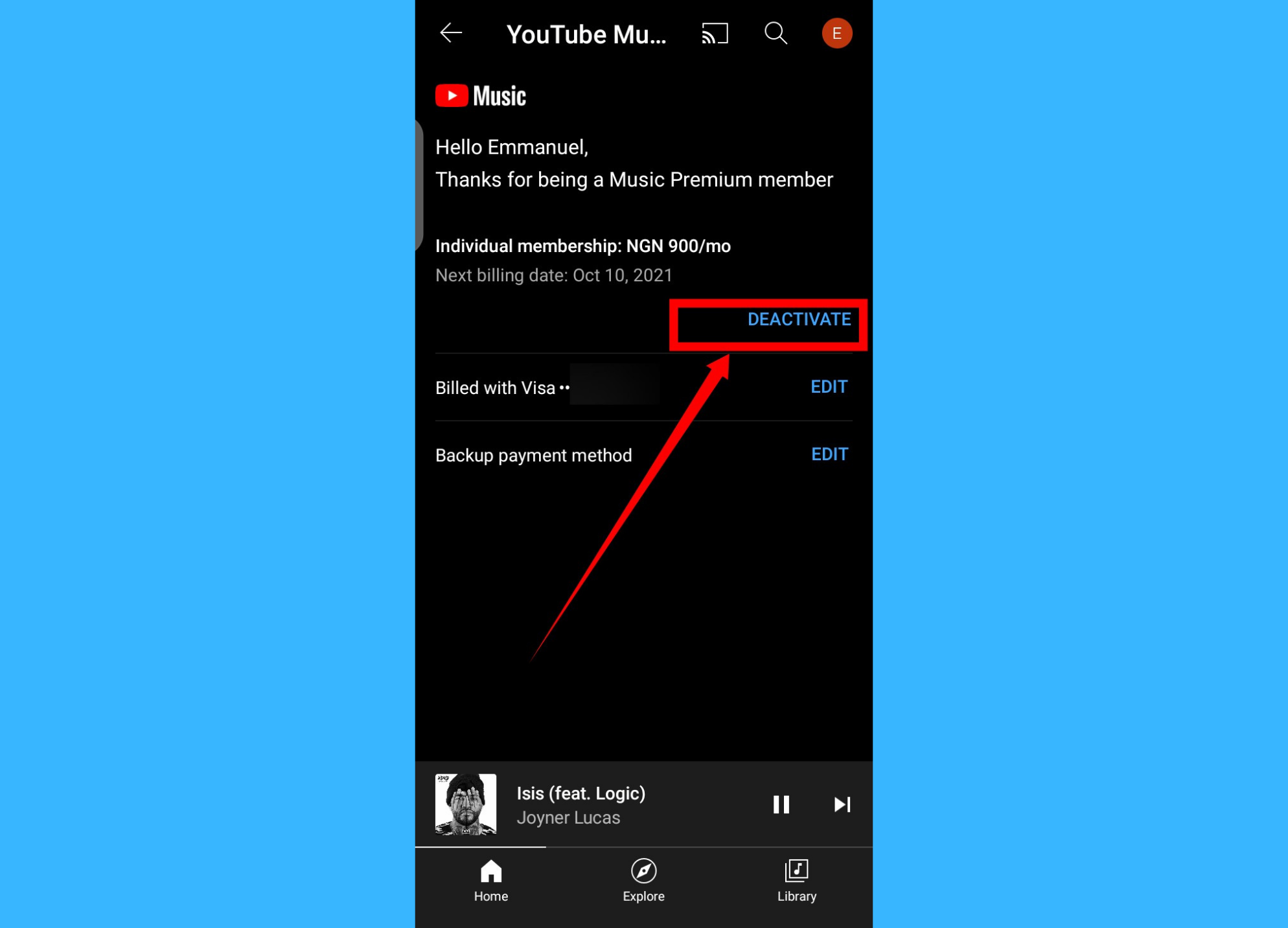The image shows a YouTube Music interface on a phone screen. The background is primarily black with white text. At the top of the screen, part of the "YouTube Music" text is truncated, displaying as "YouTube Mu...". A screencast icon and radio reception emanating from a TV are present, along with a magnifying glass icon. A user, identified as "E", is logged in, indicated by a red dot. There is also a back navigation option.

Below this, the YouTube Music logo in red is prominently displayed, followed by a greeting message: "Hello Emanuel, Thanks for being a music premier member." The membership details show "Individual Membership NGN 900 a month" in white text, with the next billing date marked as "October 10th, 2021". A blue-text option to "Deactivate" is encased in a red box, accompanied by an upward right-pointing red arrow.

Further down, the billing information includes "Bill with Visa" in white text, and an "Edit" option in blue. Additional text mentions a backup payment method next to the "Edit" option. The current track playing is "ISIS" featuring Logic, with accessible pause and forward buttons. The bottom of the screen features navigation options: Home, Explore, and Library buttons.